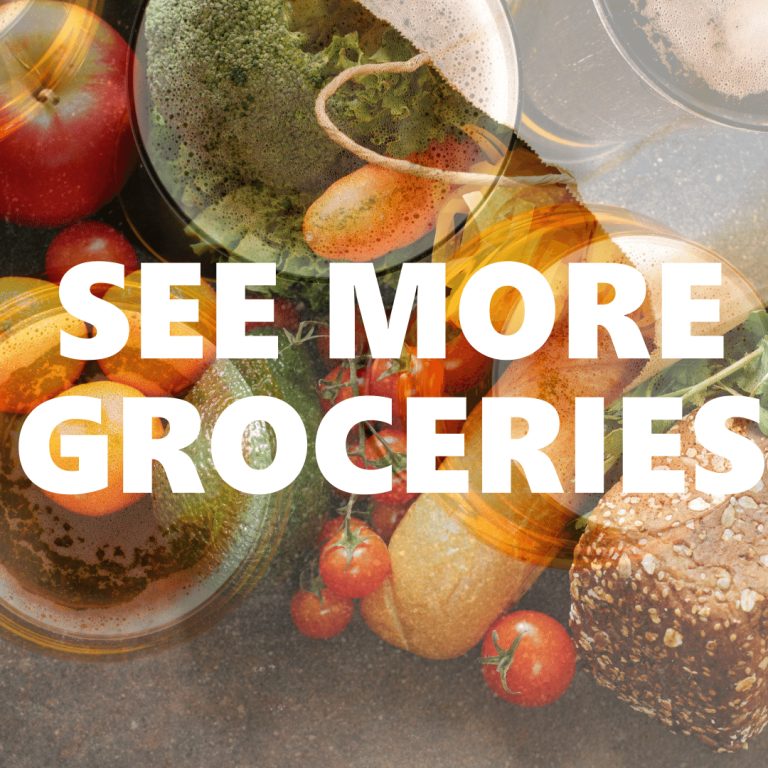The image appears to be a promotional advertisement for a grocery delivery service, depicting a variety of fresh food items. Dominating the background is a photograph of assorted groceries featuring a vivid red apple, oranges, cherry tomatoes, and two styles of bread – a pan loaf and a baguette. There are also vegetables such as green lettuce or kale and broccoli, neatly placed in container. Additional items in the image include a container that appears to have coleslaw and hints of ham. These grocery items are emerging from a grocery bag positioned at the top right of the image. Overlaying this rich display of food are the words "SEE MORE GROCERIES" in bold, white, sans-serif font, centrally located. The image has a reflective quality, possibly due to glass, adding a complex visual layer but clearly showcasing diverse, attractively arranged grocery items.